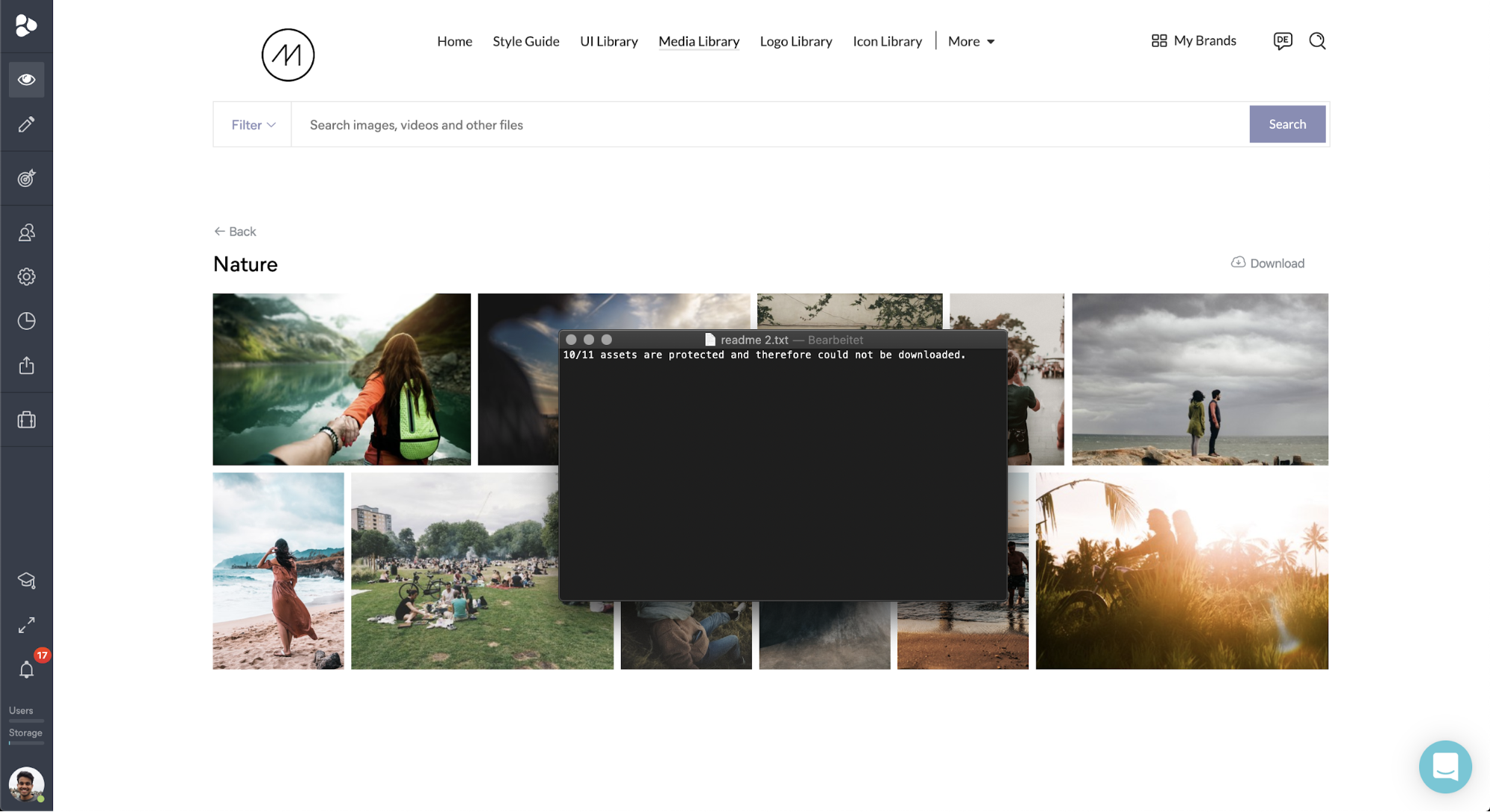**Detailed Descriptive Caption:**

The image showcases a website interface featuring a prominent circular 'M' in white on the left side, signifying the logo. At the top of the webpage, several navigation options are listed in a horizontal menu, including "Home," "Style Guide," "Library," "Media Library," "Large Library," "Logo Library," and "Icon Library," along with a dropdown arrow indicating additional options. On the right-hand side of the top menu, the text "My Brands" is displayed alongside a grid icon, a search icon, and a message icon.

A thin black vertical strip runs from the top to the bottom of the page on the right-hand side, starting with a paw print icon, followed by a series of other icons extending downward. This sidebar appears to house shortcuts or additional menu options.

In the main content area of the webpage, there is a search bar at the top labeled "Filter, search images, videos, and other files," with a blue search button at the end. Adjacent to the search bar, a small back arrow labeled "Back" is visible. Beneath the search bar, the word "Nature" is prominently displayed in a very dark black font.

The central portion of the page features a variety of images depicting people engaged in various activities, such as relaxing on a beach, standing by a river, and riding bicycles and motorbikes near water. Overlaid on this content is a semi-transparent, black-to-gray gradient pop-up. The top part of this pop-up contains text in white, but the words are not legible in the image. In the lower section of the right-hand sidebar, a red circle containing a profile picture of a white man is visible.

This descriptive caption provides a comprehensive overview of the website's interface and visual layout, capturing key details and elements that structure the user experience.